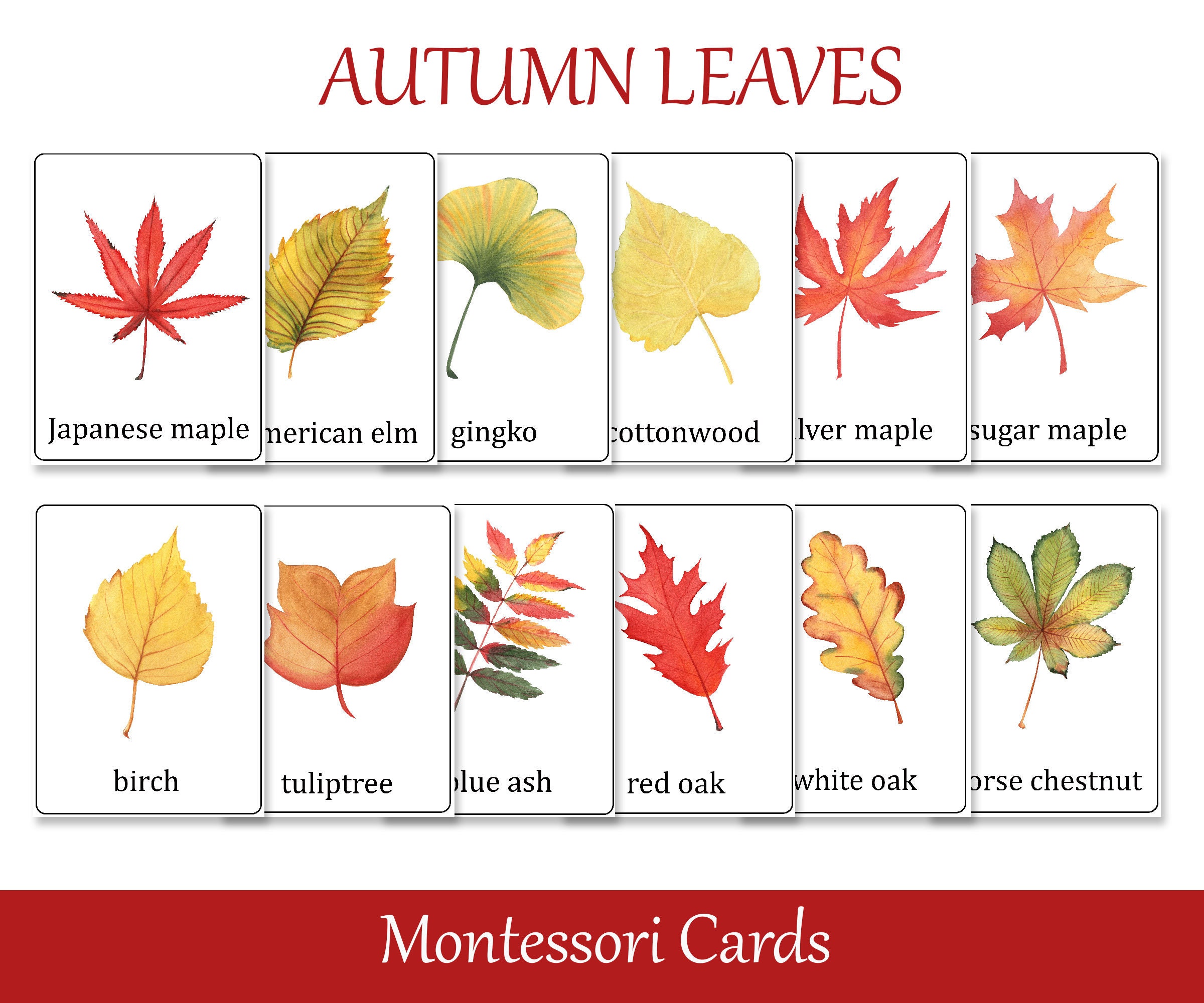The image features a chart titled "AUTUMN LEAVES" in brownish red capital letters at the top against a white background. Arranged in a slightly overlapping, layered fashion are twelve rectangular flashcards, each displaying a different type of leaf along with its name in lowercase black letters. The leaves depicted include the Japanese maple (red), American elm (green), ginkgo (yellow), cottonwood (yellow), and sugar maple, among others. On the bottom row, the leaves featured are birch (yellow), tulip tree, blue ash (tri-colored – green, yellow, and red), red oak, white oak, and horse chestnut. At the very bottom of the image, in a horizontal red rectangle with white text, it reads "Montessori cards," indicating that these might be educational flashcards.